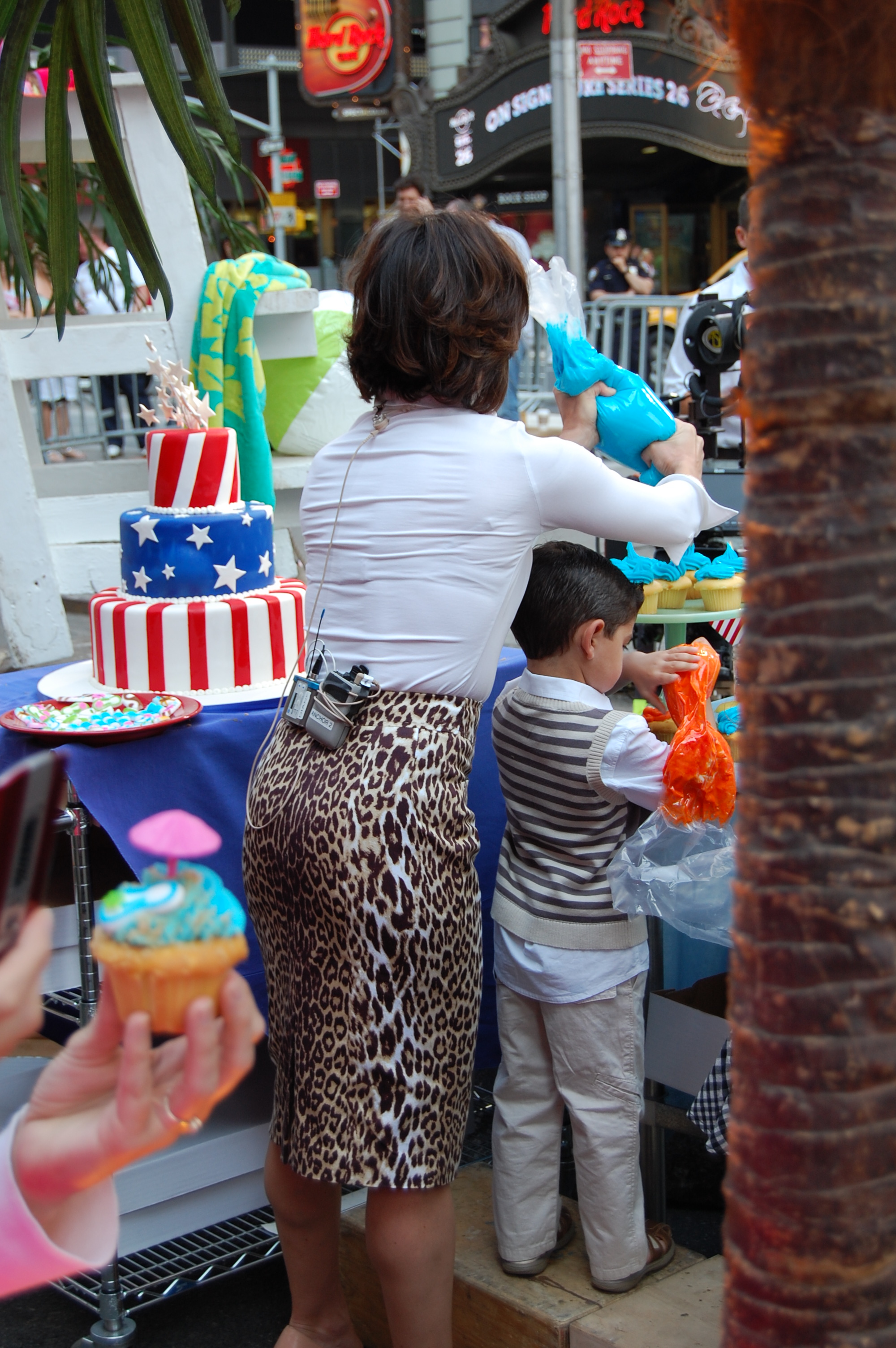In this detailed image, we see a scene centered around a woman and a young boy, both facing away from the camera. The woman sports a distinguished hairstyle with dark brown highlights over a black base, and she’s dressed in a white long-sleeve shirt paired with a form-fitting leopard print pencil skirt. Attached to the back of her skirt is a microphone, suggesting she might be involved in a speaking engagement or presentation. 

In front of her, a neatly groomed boy stands with a head of well-combed hair. He is dressed in a white dress shirt beneath a striped brown and white vest, which he pairs with white pants. Both the woman and the boy are engrossed in an activity, each holding a bag of frosting—hers blue and his orange—as they work together to decorate cupcakes.

To the left of this duo, there’s an eye-catching three-tiered cake adorned in a red, white, and blue theme. The bottom tier features red and white stripes, the middle tier is blue with white stars, and the topmost tier returns to the red and white striped pattern. A plate nearby implies that the cake might be ready to be served soon.

In the lower-left corner of the frame, a hand appears, palm facing up, emerging from the edge of the photo. This hand, with a ringed finger and a bit of a sleeve showing, is holding a vanilla cupcake topped with blue icing and a small pink decoration protruding from the top. This touch adds another layer of detail and interest to the scene.